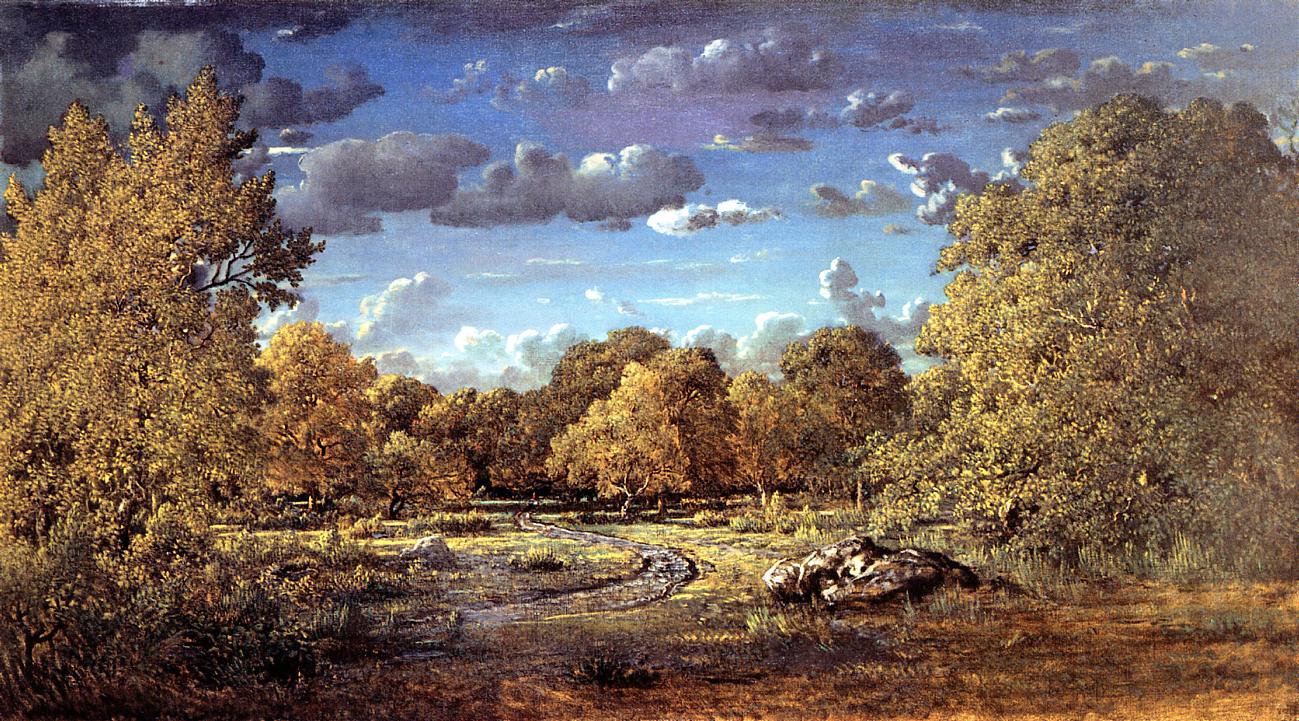This painting captures a vibrant, picturesque nature scene centered around a winding river that curves like a backward 'C'. Tall trees with yellowish-golden leaves frame both sides of the canvas, their foliage dense and full. Towards the horizon, more leafy trees dot the landscape, adding depth to the scene. The ground is covered with varied shades of green grass, transitioning to light brown in the foreground, dotted with bushes and occasional rocks. A notable large boulder sits just right of center in a grassy field that slopes gently towards the stream. The sky above is a lively blue, punctuated by puffy white clouds and occasional darker patches, suggesting a mix of sunny and cloudy weather. The overall artwork strikes a balance between cartoonish elements and photorealistic vibrancy, making the colors pop and the scene come alive. No creatures or people are visible, giving an untouched, serene quality to this wilderness vista.